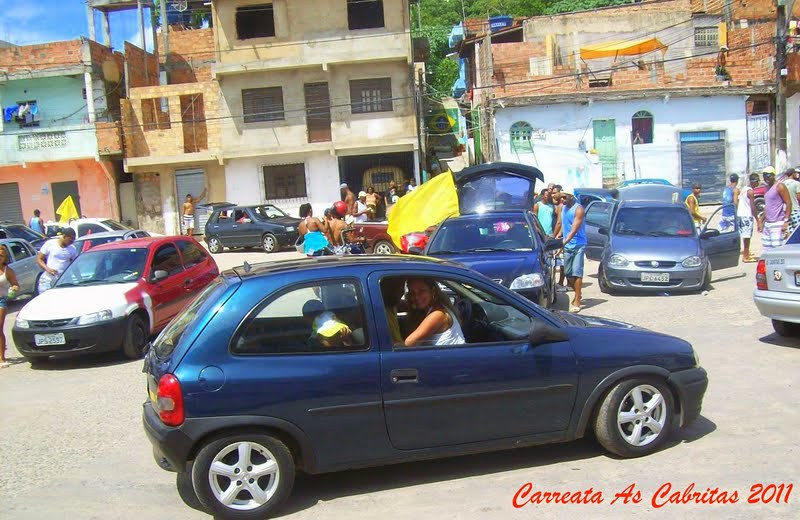The image depicts a bustling scene, likely a busy marketplace or a communal event. In the foreground is a blue, two-door hatchback with two people inside. The driver is not clearly described, but the female passenger, wearing a white sleeveless blouse, gazes directly at the camera over her left shoulder. Surrounding the car are various other vehicles parked haphazardly, some with doors open and trunks lifted, signifying an active environment. Several individuals are seen exiting their cars and walking towards a set of buildings in the background.

The backdrop consists of three buildings: a two-story house on the left, a three-story possibly apartment building in the center (notable for a visible car garage), and a single-story white adobe structure with a distinctive canvas tent setup on top. Beach umbrellas and women carrying beach bags suggest the possibility of a nearby beach. The overall scene hints at a modest, even impoverished community, signified by the partially constructed or repaired buildings. The photograph is marked with red cursive text at the bottom right corner, stating "Carriata as Cabritas, 2011".